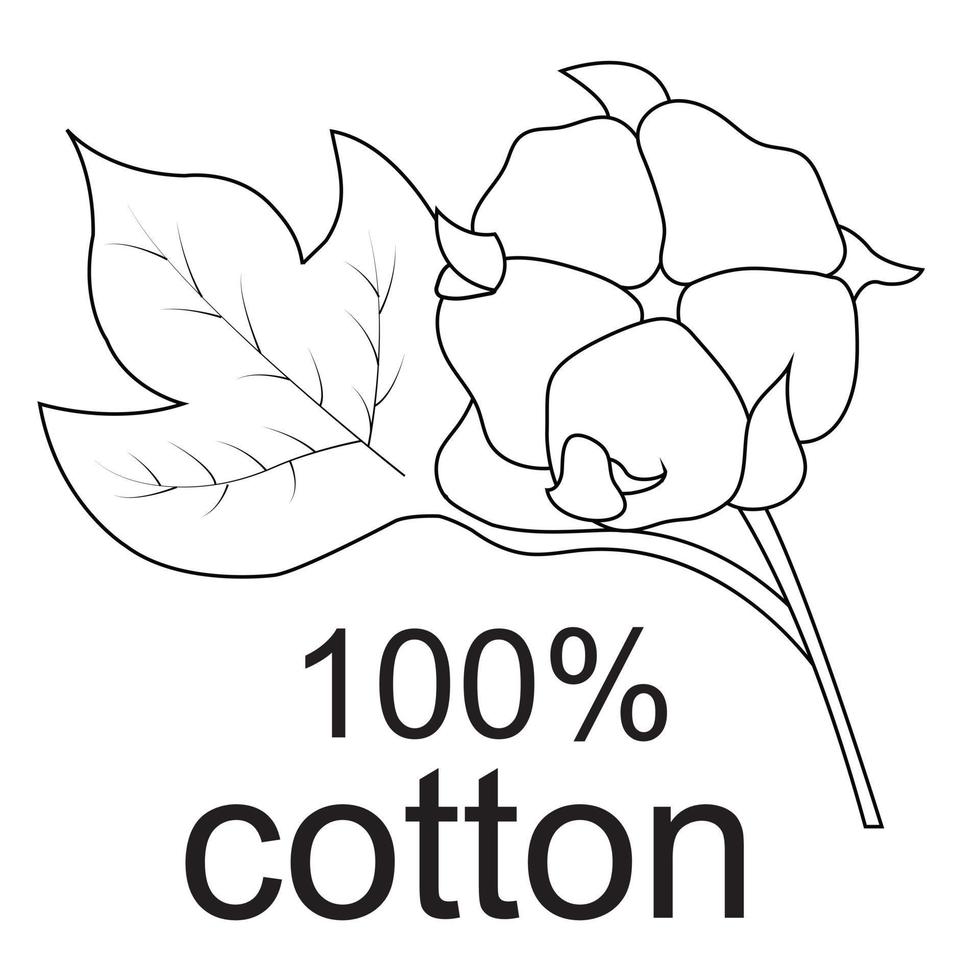The image is a black and white graphic without a border, featuring a line illustration of a cotton plant in the center. On the lower right, a stem extends upwards and curves toward the middle, branching off in a curved line to the left forming a leaf, and further branches right into the cotton flower. The leaf on the left side has three pointed, curved sections with visible veins. On the right side, there is a cotton flower with five petals and smaller parts visible between them. Below the illustration, centered at the bottom, there are two lines of bold black text: "100%" on the top line and "cotton" in lowercase letters on the second line. The background is plain white, emphasizing the detailed line work of the graphic.